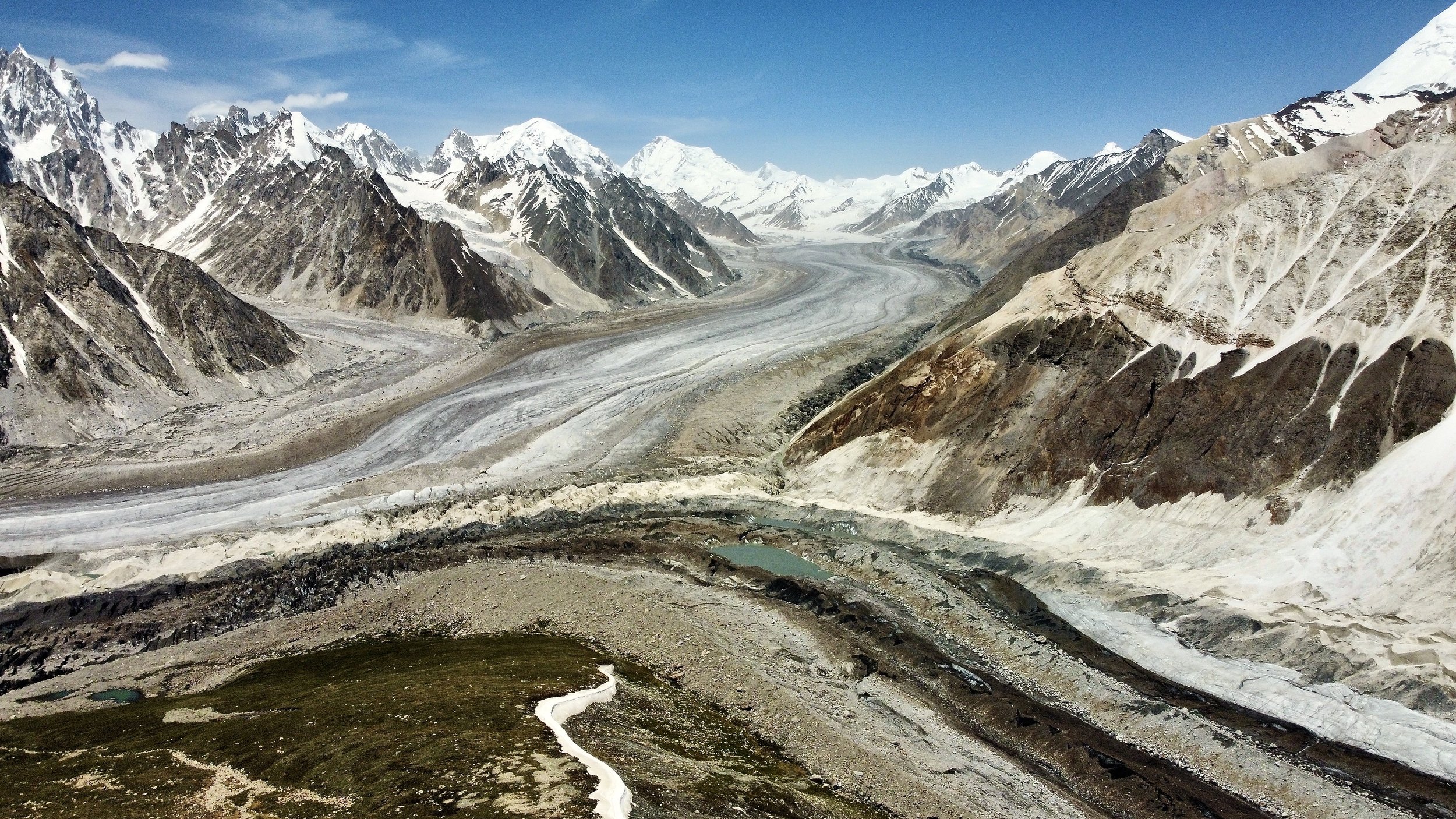In this daytime outdoor scene, a winding road traverses through a rugged mountain landscape blanketed with snow. The road starts at the bottom left, winds toward the center, then ascends and weaves back and forth. In the far distance, the mountains are sharply peaked and heavily snow-covered, devoid of any vegetation. The sky above is predominantly blue with some scattered clouds on the left. On the far right, an even taller, predominantly brown mountain range rises, capped and streaked with snow. To the left side, the mountains feature gray rocky formations also lined with snow. In the center of the image, a green-colored puddle sits in a section of the road that curves to the right before continuing downward to the bottom right. The ground around the road is a mix of light brown and gray, with patches of ice visible. A strip of white runs alongside the left side of the road, swerving up and to the left before stopping beside a pile of gray dirt, creating a natural barrier next to the road.